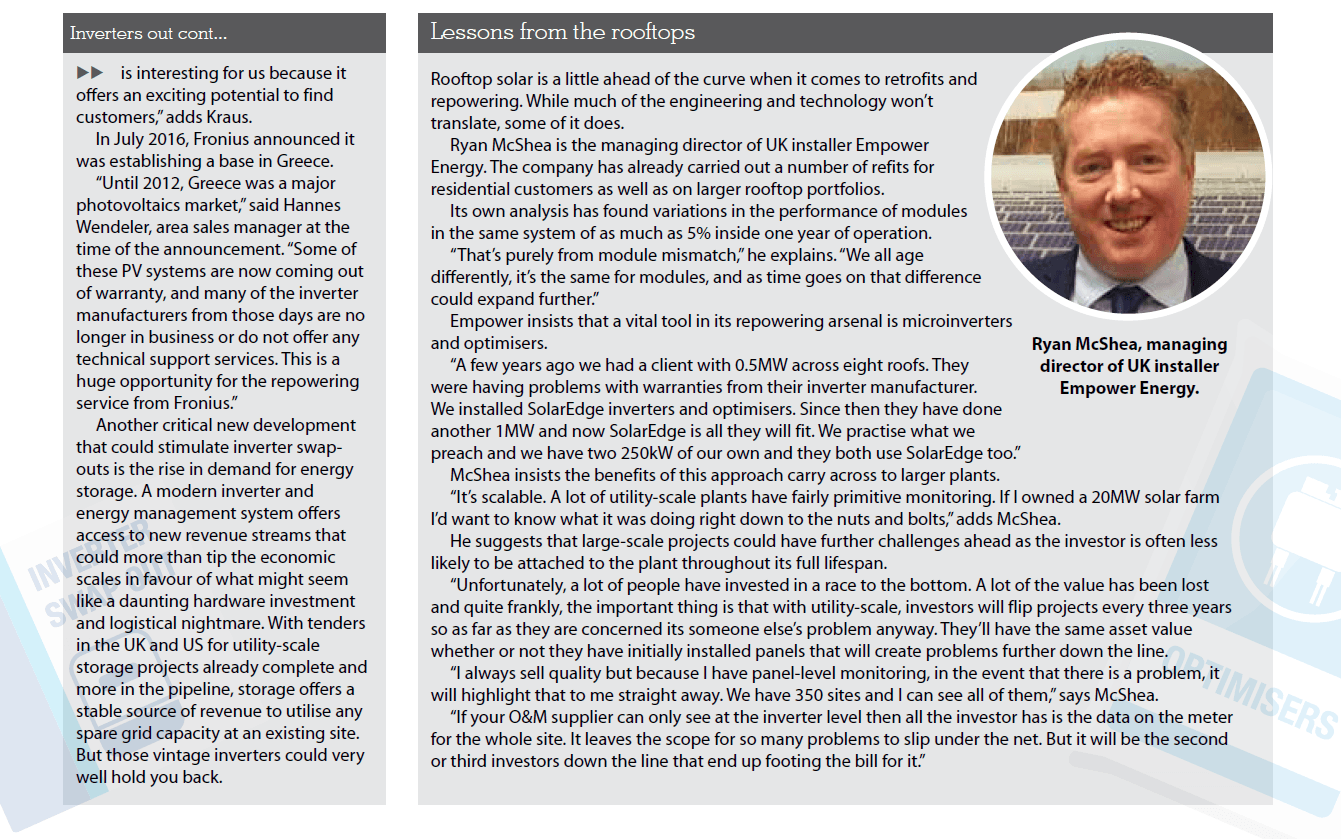The image appears to be a page from a textbook, divided into two distinct sections. The first section is a narrow box positioned at the top of the page, featuring a gray banner with the text "Inverters (continued)...". The second box is significantly larger but of the same length, also topped with a gray banner that reads "Lessons from the Rooftop".

On the far right side of the page, there is a circular, white-outlined photograph of a middle-aged white male, presumably in his 40s, standing in front of a solar panel farm. He is dressed in a suit with a tie adjusted firmly around his neck. He appears to have reddish hair. Below the photograph, a caption identifies him as "Ryan McShay, Managing Director of UK Installer and Power Energy."

The larger section of text delves into the subject of rooftop solar, suggesting that it is slightly ahead in the area of retrofitting and repowering compared to other sectors. Although much of the engineering and technology might not be directly transferable, some elements do apply. The text highlights that Ryan McShay’s company has executed numerous refills for both residential clients and larger rooftop portfolios. The content mainly consists of multiple paragraphs focusing on Ryan McShay and his company’s work and expertise in the field of rooftop solar energy.